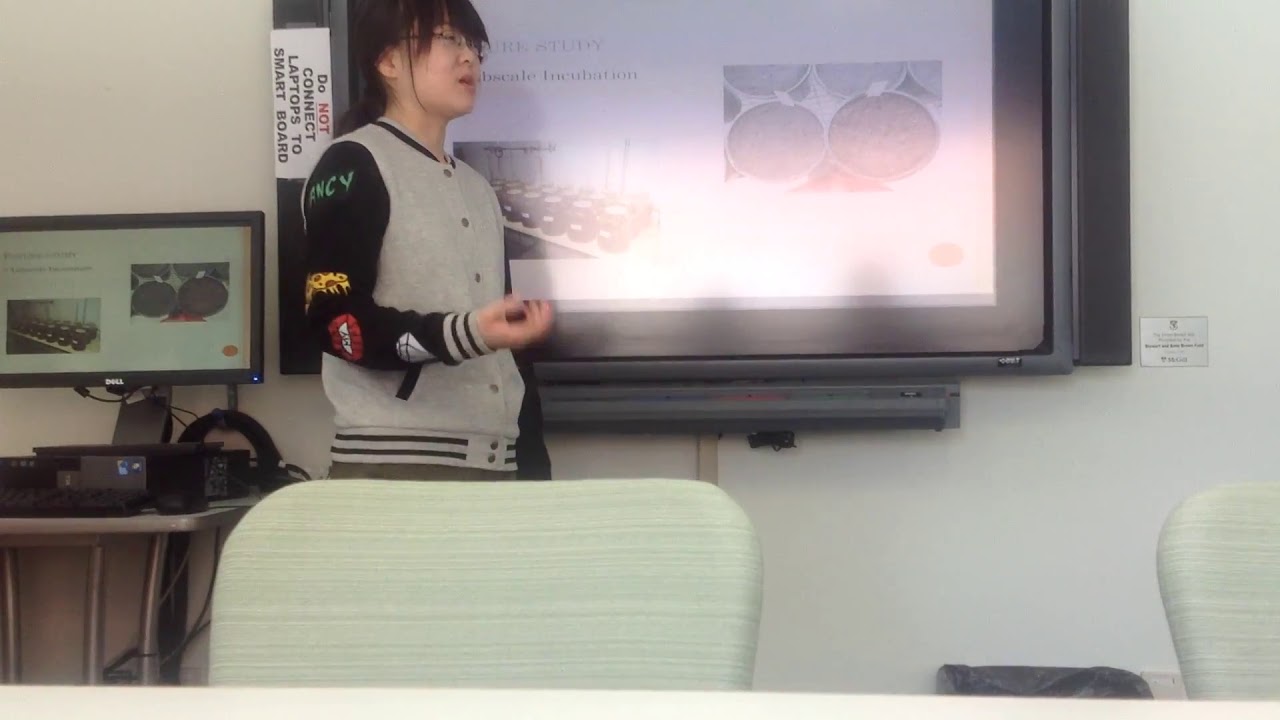In the image, an Asian woman with straight, shoulder-length black hair featuring bangs and a partial ponytail, wears clear eyeglasses with black frames. She stands to the center-left, facing right, next to a bright screen or TV mounted on a white wall. The screen, which also has significant glare, displays what appears to be a presentation slide with a white background, text, and two images—though most details are obscured by glare and her position. To the left of the woman is a desk topped with a black computer monitor, which mirrors the slide on the TV. The monitor has a black bezel and sits above a black desktop tower. A keyboard and mouse are also visible on the light gray desk. The woman's outfit includes a gray and black button-up jacket adorned with various patches; green letters ending in "C-Y" on the upper sleeves, and additional patches in yellow, brown, red, white, and another white one near her elbow. Black stripes accent the collar area and base of the jacket. Her right arm appears blurred, suggesting motion. In the foreground, a light mint-green chair with horizontal lines is partially visible, with its top backrest showing prominently. Another similar chair is cropped in the bottom right corner. To her right, a sign on the wall warns, in predominantly black text with a red "not," against connecting laptops to a smartboard.